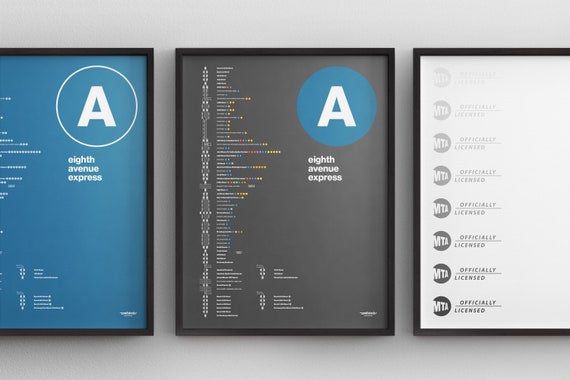This photograph showcases three framed prints, each displayed side-by-side on a plain white or very light gray wall. The frames are thin and black, providing a minimalist aesthetic. The first print on the left has a dark blue background and features a large white capital 'A' within a thin white circle positioned at the top right. Beneath this, it reads "8th Avenue Express" in white letters. Some additional text is visible but not clearly legible. The second print in the center has a similar design but with a gray background. The 'A' is in the same position but within a teal circle, again above the words "8th Avenue Express." This print also contains small, multicolored letters—blue, yellow, red, and green—that are difficult to decipher. The third print on the right departs from the bold 'A' theme and instead has a white background. It repetitively features the phrase "officially licensed" beside small, round MTA logos, running from top to bottom. The grayscale and MTA branding suggest that these might be official transit-related prints, possibly preview images showing how they would appear framed on a wall.